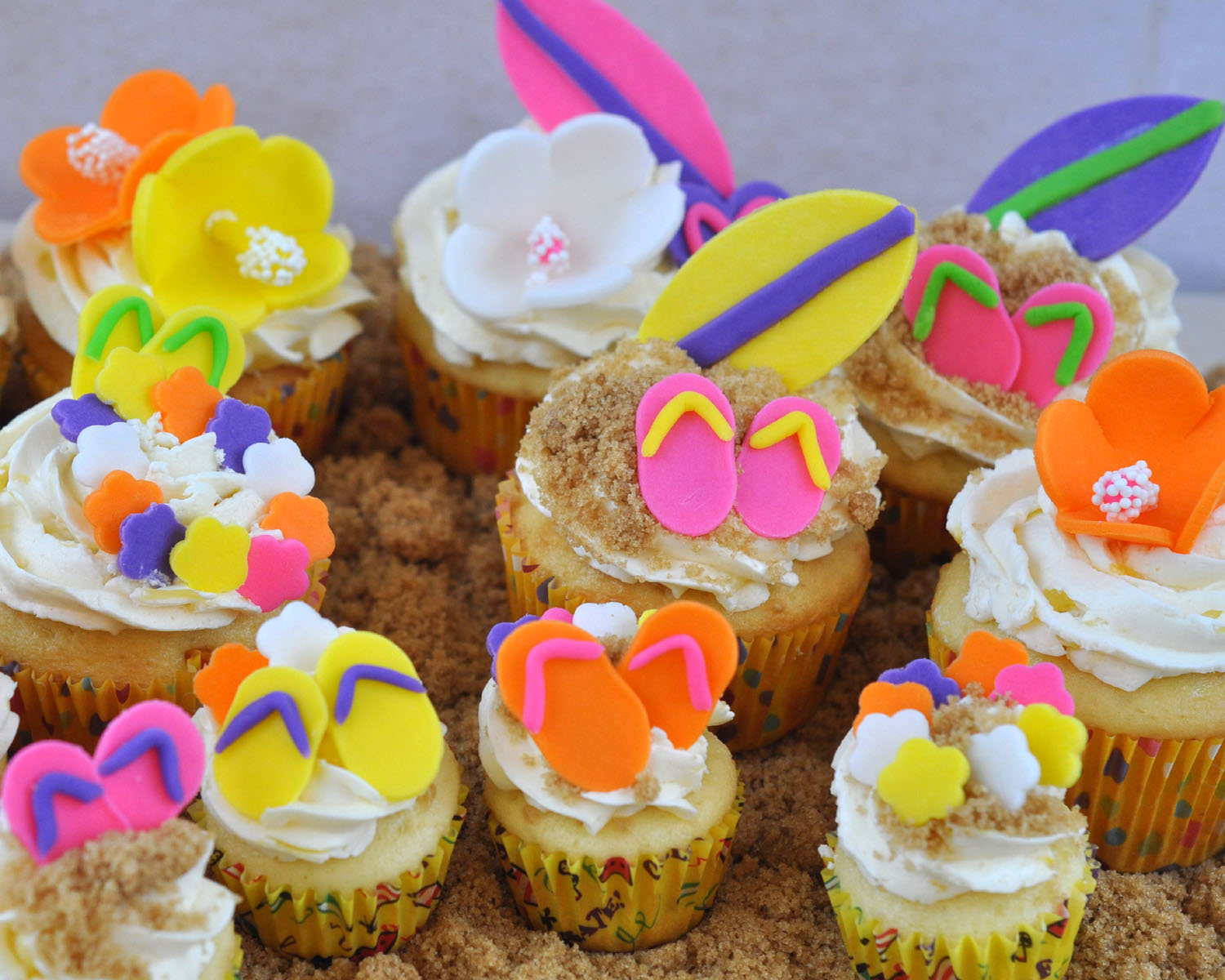This color photograph showcases an array of cupcakes meticulously designed with a beach motif. The cupcakes, seemingly made from yellow cake batter, are adorned with white frosting and set atop what resembles brown sugar, mimicking the appearance of beach sand. Each cupcake features various edible decorations crafted from fondant, including flip-flops with contrasting colored thongs, surfboards, and tropical flowers such as orange, yellow, and white orchids. Scattered among these are star-shaped petals and other tropical-themed accessories. The decorations are vivid, with splashes of yellow, pink, blue, orange, white, and green. The cupcakes are organized in rows, with the closest row extending off the bottom and left edges of the image, revealing intricate details like pink hearts, yellow ovals with blue arrows, and white icing. The middle row consists of three regular-sized cupcakes with a variety of rounded, bulging shapes and some with surfboard-like designs. The scene is set against a gray background, lending a neutral contrast to the vibrant, beach-inspired treats.